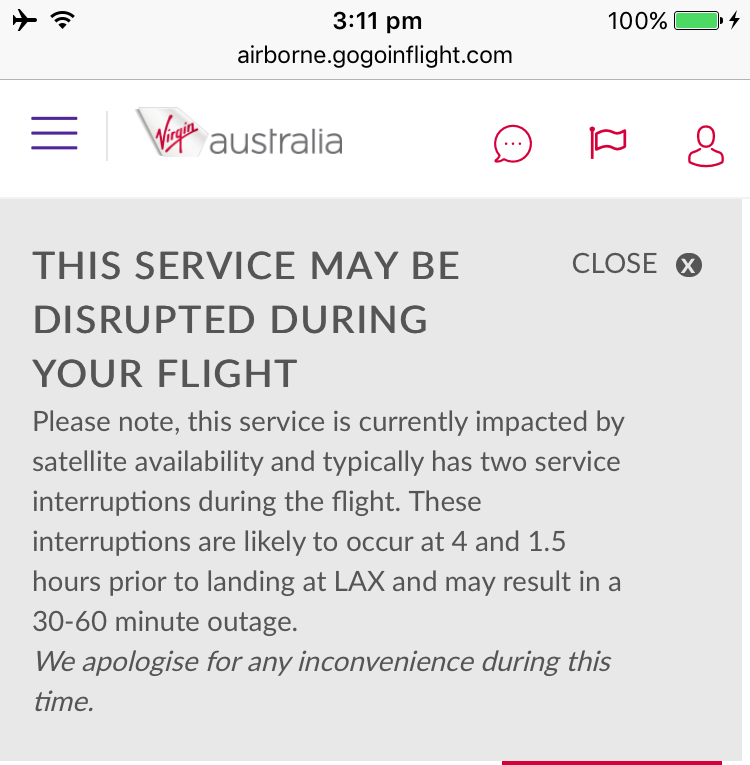This screenshot captures a webpage on an inflight Wi-Fi service. The top of the image features a grey background with an airplane icon and a Wi-Fi symbol. Centered prominently is the current time displayed as 3:11 PM, with the URL "airborne.gogoinflight.com" positioned just below it. To the right, the battery icon is fully green with a small lightning bolt, indicating a 100% charge.

Below the header, a white banner contains three horizontal purple lines aligned vertically, followed by the word "Virgin" in red text next to "Australia." Adjacent to this, a text bubble icon with an ellipsis inside, a red flag, and a silhouette of a person’s head and shoulders are visible.

A grey banner beneath this section reads: "This service may be disrupted during your flight." Next to it, a small circle with an 'X' offers a closing option for the notice.

Further down, a detailed message provides additional information: "Please note this service is currently impacted by satellite availability and typically has two service interruptions during the flight. These interruptions are likely to occur at four and one and a half hours prior to landing at LAX and may result in a 30 to 60 minute outage. We apologize for any inconvenience during this time."